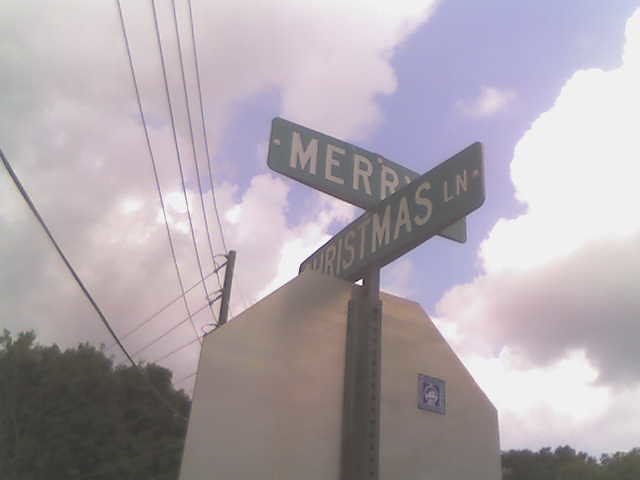Under a vibrant blue sky, a mix of dark grey and light grey clouds float lazily. Crisscrossing the scene, several electric lines stretch between sturdy poles, adding a sense of structure to the atmosphere. On both the left and right peripheries of the image, the lush green foliage of tall trees frames the composition. In the foreground, the metallic silver back of a stop sign gleams, adorned with a small blue sticker that reads "Merry Christmas Lane" in white lettering. The sign's pole features a textured design with small dots. The contrasting colors and elements combine to create a picturesque and tranquil urban landscape.